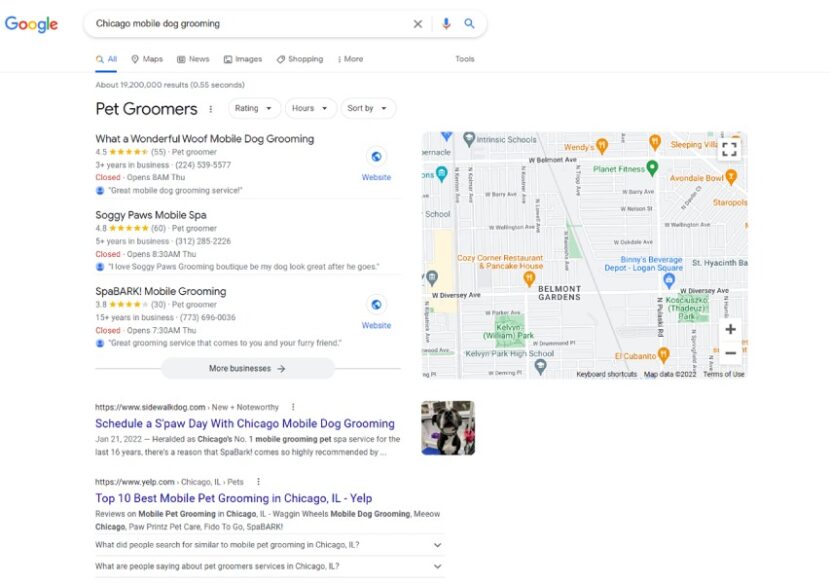A Google search for "Chicago mobile dog grooming" is displayed, showing a list of pet groomers in the area. At the top of the search results, three prominent mobile grooming services are featured: "What a Wonderful Wolf Mobile Dog Grooming," "Soggy Paws Mobile Spa," and "Spabark Mobile Grooming." Each listing indicates their status as currently closed, with opening times on Thursday morning—8:00 a.m., 8:30 a.m., and 7:30 a.m., respectively. 

On the right side of the screen, a map highlights various locations with pins, presumably marking the addresses of these mobile grooming services. Below the top three listings, there's an option to explore more businesses. Each grooming service also includes customer reviews, providing insight into their quality. Additionally, links to two articles are visible: one for scheduling a spa day with Chicago mobile dog grooming and another listing the top 10 best pet grooming services in Chicago, Illinois.